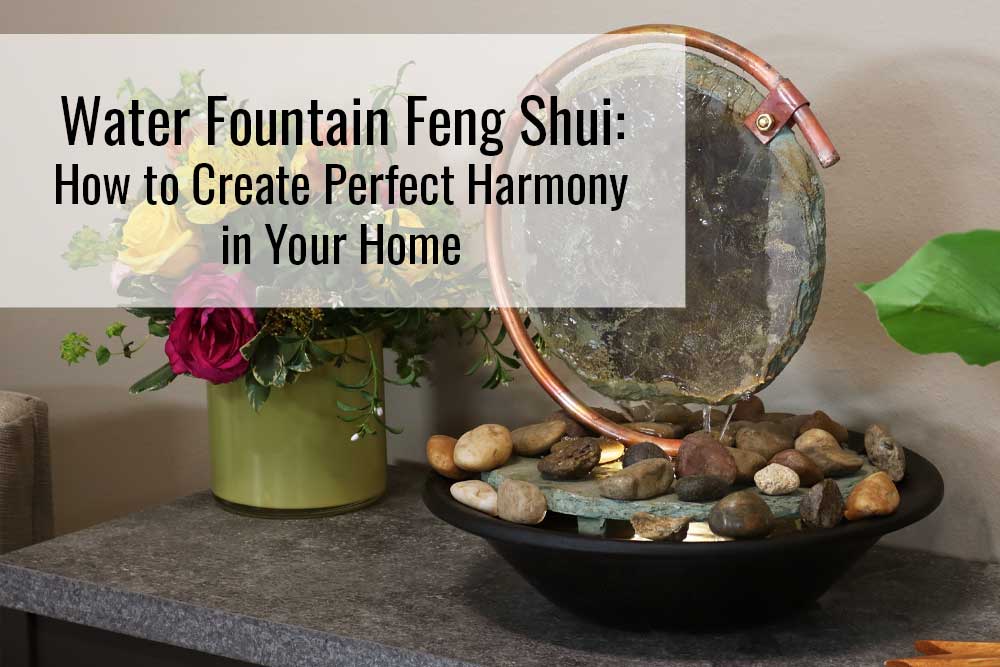The image depicts a staged scene promoting a water fountain for sale, emphasizing its Feng Shui benefits for creating harmony in a home environment. Central to the image is the water fountain, featuring a black bowl filled with small rocks and a stone apparatus resembling a round mirror, encircled by flowing water. The design incorporates both flat and cascading arrangements of stones. Positioned to the left of the fountain is a flower arrangement in a green vase, containing white, red, and yellow roses, along with green leaves. The scene is set on a table and accompanied by text overlay reading, "Water Fountain Feng Shui: How to Create Perfect Harmony in Your Home." The overall composition showcases the interplay of water, stones, and flowers, enhanced by shadows cast on the wall.